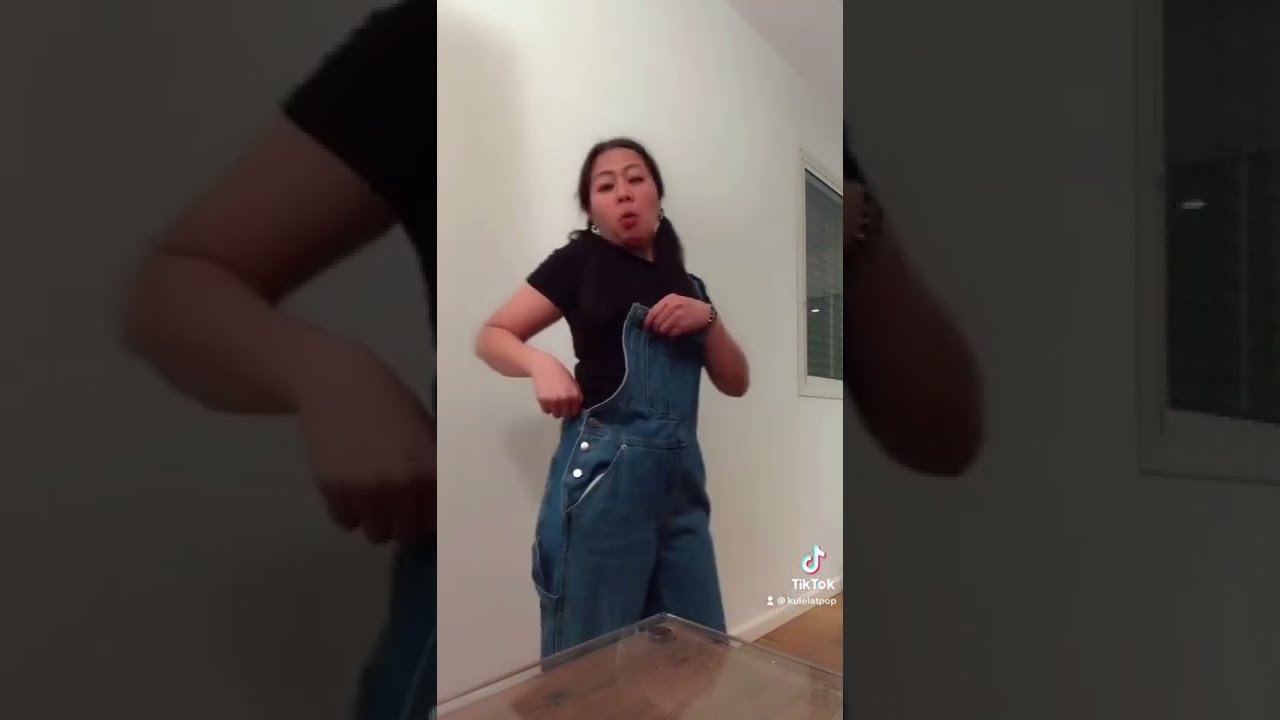The inside of a house frames the scene, featuring a young woman who appears to be of Asian descent. She has slightly closed eyes and a playful, energetic expression on her face as if she's making a funny gesture. Her black hair contrasts with her light, although slightly darker skin tone, distinguishing her from being Caucasian. She's dressed in a black t-shirt under a pair of light blue jean overalls, but one of the shoulder straps is undone, giving the impression she's either in the process of fixing it or demonstrating a unique styling method, likely for her TikTok channel. In the background, a white wall, wooden floors, and an open window with blinds can be seen. The chic aesthetic is complemented by a sleek, glass-top table on which a camera is perched, capturing her creative content. The image is slightly blurry, but the vibrant energy of the scene is unmistakable. Overlaid symbols and text in the bottom right reveal this is a TikTok video, with the profile handle '@KulapPop,' suggesting she's a popular content creator on the platform.